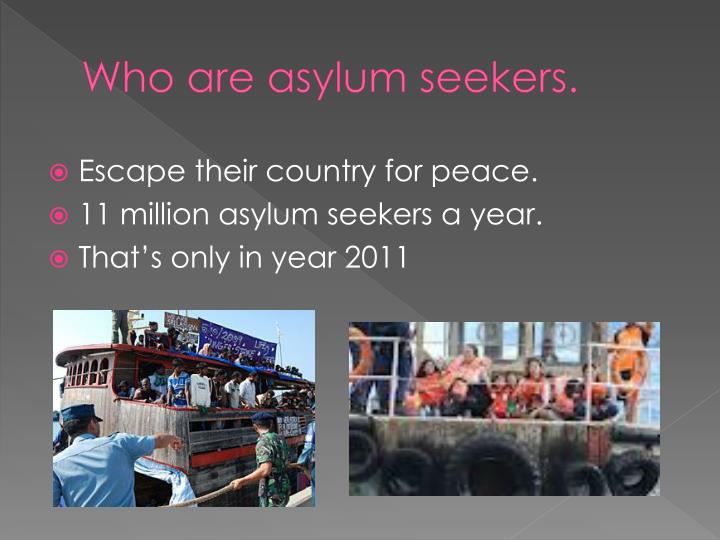The image is a detailed and impactful informational poster. At the top of the poster, bold red-pink text reads "Who Are Asylum Seekers?" against a dark gray background. Directly below, three pink bullet points with accompanying white text state: "Escape Their Country for Peace," "11 Million Asylum Seekers a Year," and "That's Only in Year 2011." The lower section of the poster features two landscape-oriented color photographs. The photo on the bottom left shows a crowded boat filled with asylum seekers, with some officials standing nearby. The photo on the right depicts another boat with people, including children, sitting down, and tires hanging from the sides. Despite the poor quality and blurriness of the images, the urgency and dire circumstances of the asylum seekers are clear. The poster combines photographic realism with graphic design to vividly communicate the plight and statistics of asylum seekers.